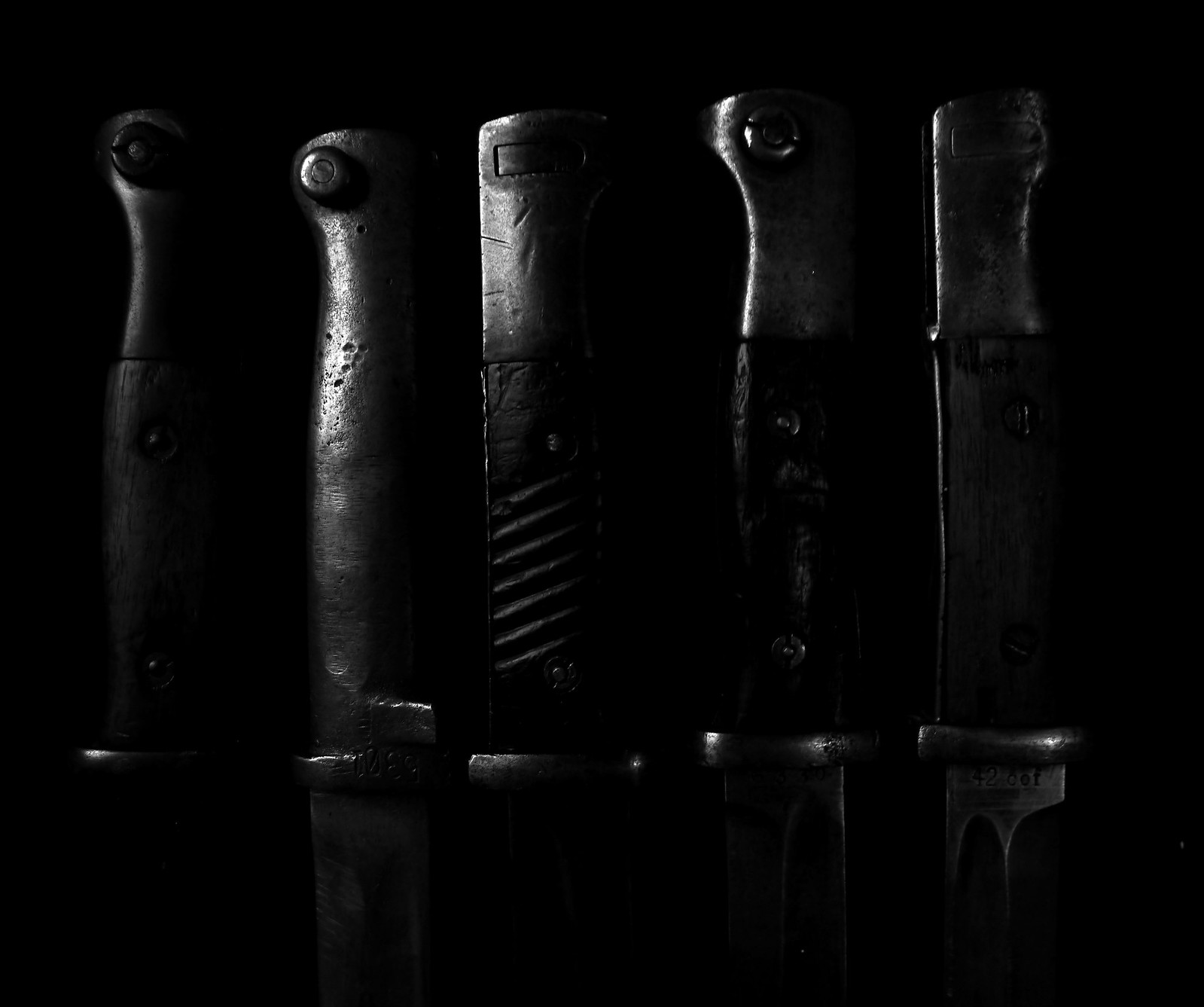The image depicts a close-up of five knife handles, each featuring unique and intricate details, set against a black background with minimal lighting. The two handles on the left have large black screws at the tops, contributing to their rugged appearance. The middle handle stands out with its black textured grip, while the handle to the right of it is embellished with numerous rivets. The far-right handle showcases a somewhat flanged hilt. Each knife is equipped with a thin ring guard near the base, and their metal bodies gleam faintly in the dim lighting, suggesting they are made of metal. The background’s darkness makes it challenging to discern the blades clearly, yet the knives' distinctive characteristics and orderly arrangement are evident, set against the deep black backdrop.